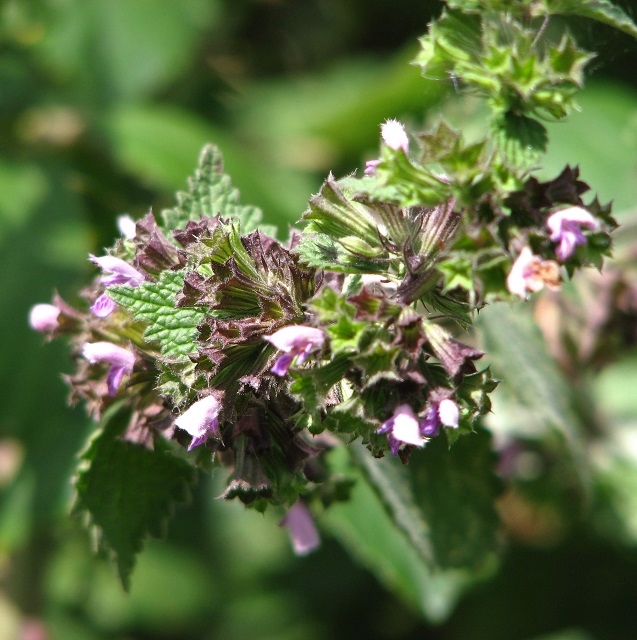This close-up image captures a flowering herbaceous plant or shrub, possibly in the wild. Dominating the frame, the plant showcases bilabial flowers that are very small, with a light pinkish-purple or white-purplish hue. The flowers appear to be emerging from spiky, still-opening leaves or petals. Additional details reveal some of the flowers are in bloom, others are budding, and a few are browning, indicating different stages of the flowering process. The leaves, small and green with a texture that resembles those of the pelargonium species, intermingle with the flowers. Interestingly, there's a light red or pinkish growth on the leaves near the flowers. The backdrop consists of blurred greenery, potentially more foliage from the same plant, providing a rich, natural context to the sharply focused flowering section that occupies approximately 25 to 33 percent of the image.